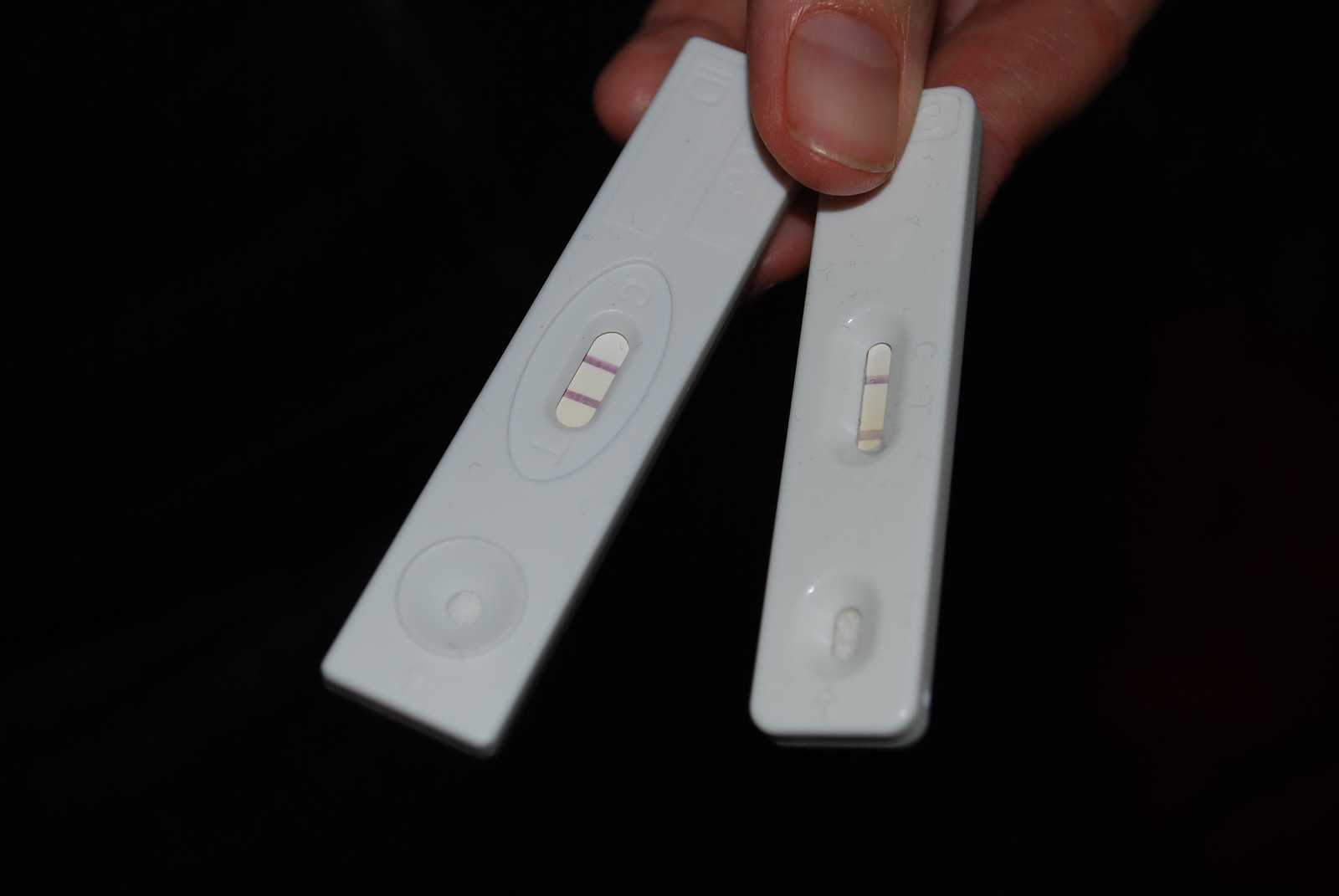In the image, set against a stark black background, a hand is partially visible holding two differently-sized white plastic objects that appear to be pregnancy tests. The objects are approximately three inches in length. Both devices feature indentations and strips that show results. The first test has an indented circle at the bottom, followed by an oval-shaped indentation in the center, containing a white strip with two parallel purple lines, indicative of a positive result. The second test is slightly shorter. It also has an indented circle at the bottom, reminiscent of a tiny button, and an oval indentation in the center. Like the first, the central white strip on this test also displays two parallel purple lines. The image appears to capture the moment of verifying a pregnancy with two different tests, ensuring accuracy in the positive outcome.